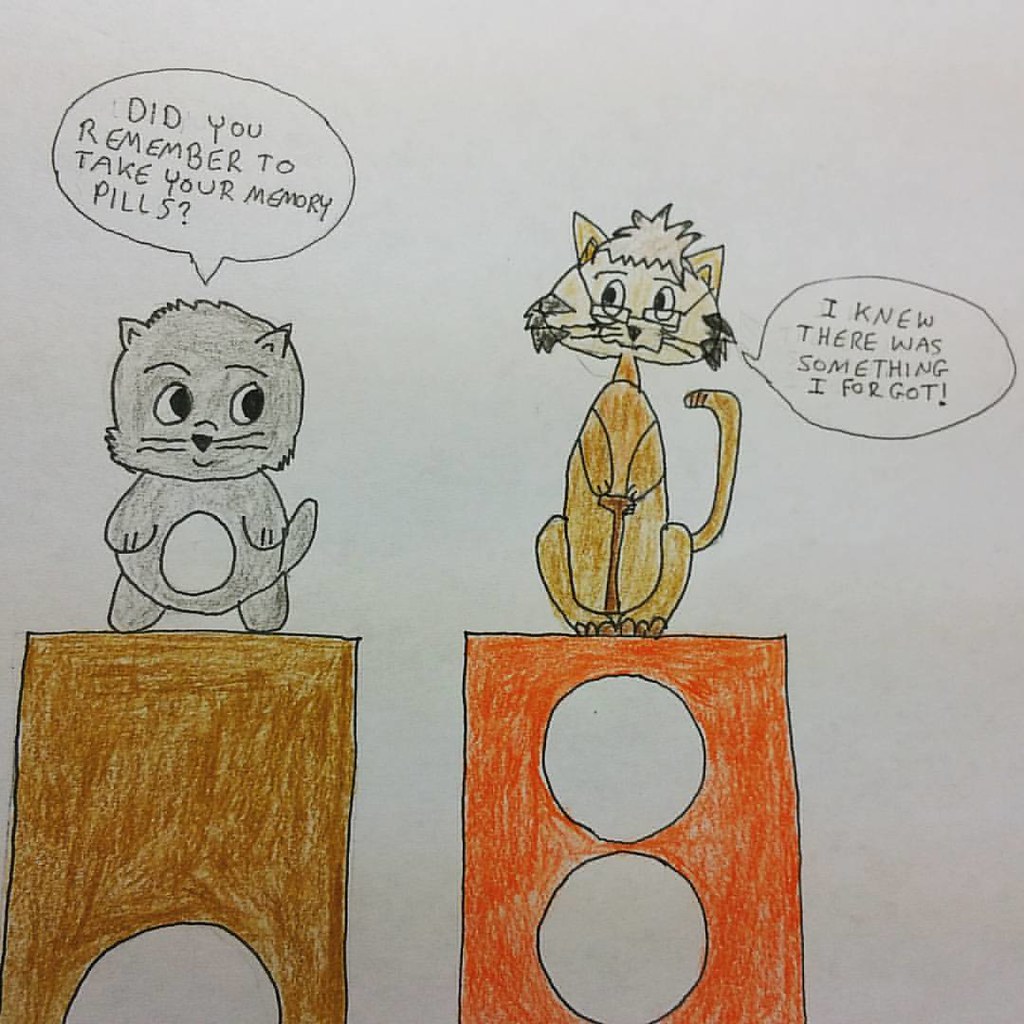This image appears to be a hand-drawn comic on white or light gray paper, possibly created by a child due to the informal handwriting style. On the left, there is a small, plump gray cat with a round white belly, standing on a brown stand with a small arch or circular opening at the bottom. Its ears are pointed and situated on top of its head, giving a horn-like appearance. The cat's eyes look to the right, and it has a text bubble above it reading, "Did you remember to take your memory pills?" 

To the right, there is another stand, orange in color with two white circular holes vertically aligned in the middle. Sitting on this stand is a brownish-beige cat with white and black fur patches on its cheeks. This cat, which has a tuft of hair on its head and wears glasses, appears older and thinner. Its ears are pointed and placed on the sides of its head. The cat also holds a cane and has a text bubble next to it saying, "I knew there was something I forgot." The entire drawing is created using colored pencils or crayons.